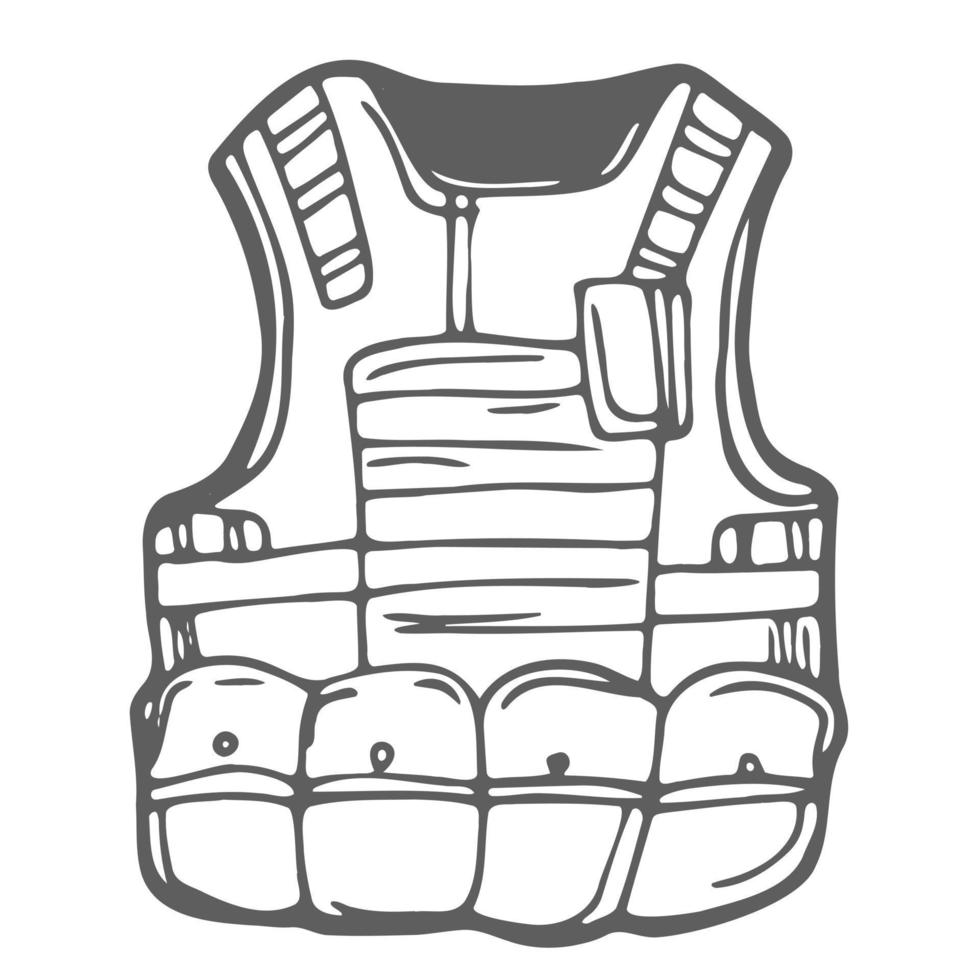This black-and-white drawing depicts a detailed tactical vest, possibly intended for military or police use, characterized by its sleeveless design with shoulder straps offering additional support via smaller attached straps. The top right corner features a small pouch, while the midsection includes a chest and stomach plate for added protection. An encircling white belt is positioned about two-thirds down the vest, visually segmenting the design. The bottom section is lined with four distinct pouches, each equipped with buttons, indicating their potential for storage. The entire illustration appears lightweight and tactically efficient, while also holding a cartoony aesthetic.